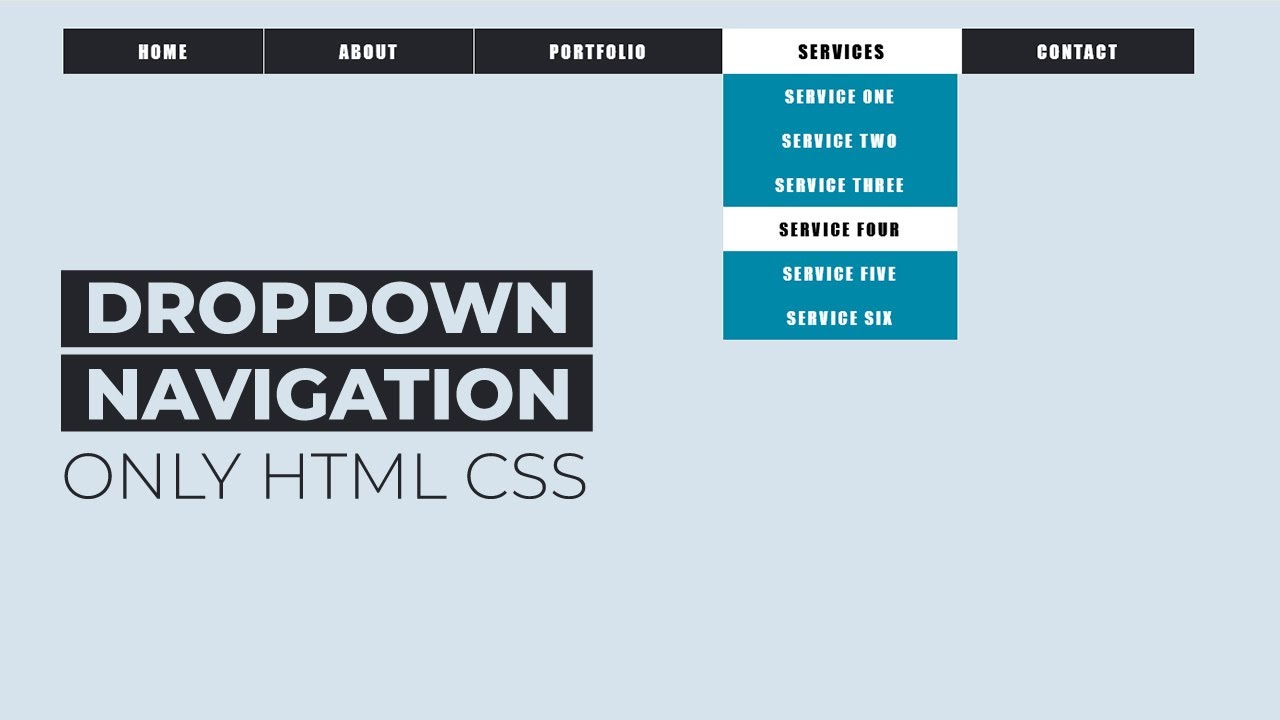### Website Screenshot Description

The image captures a screenshot of a website with a background color of light bluish-gray. At the top of the page, there is a black menu bar containing five primary sections. From left to right, these sections are labeled: Home, About, Portfolio, Services, and Contact. 

The "Services" section differs from the others as it has a white background, indicating it is a drop-down menu. When expanded, the drop-down menu reveals a list of six services. The background of the drop-down menu is teal. The services listed are:
- Service 1
- Service 2
- Service 3
- Service 4 (highlighted in white)
- Service 5
- Service 6

Beneath the menu bar, there is a section of text enclosed within black boxes around each individual word. The boxed text reads "drop-down and navigation." Directly below this text, there is another line of text that states "only HTML CSS," presented in a monospaced font. 

The overall design of the website is clean and structured, with a clear distinction between the sections and interactive elements.